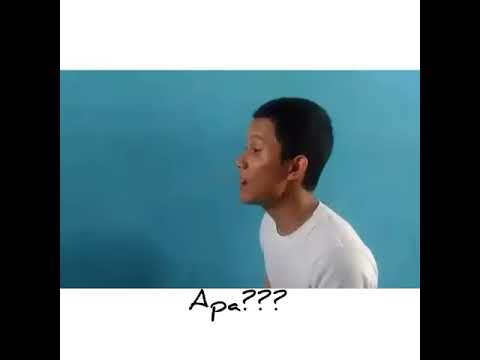The image depicts a young man with dark brown skin and short black hair, standing against a solid blue wall with an aqua-like hue. He is wearing a plain white t-shirt and is positioned on the right side of the frame, looking to the left. The view captures him from the top of his shoulders upwards, showing his torso, neck, and head. His mouth is open and his eyes are wide with raised eyebrows, giving a sense of expression. 

There is a shadow on the wall to the left of his head, likely cast by him due to the light positioning. Surrounding the main image are white bars at the top and bottom, and thin black vertical bars on either side. At the bottom of the image, on a white background, there is text in a handwriting-style font that reads "APA???" in black.